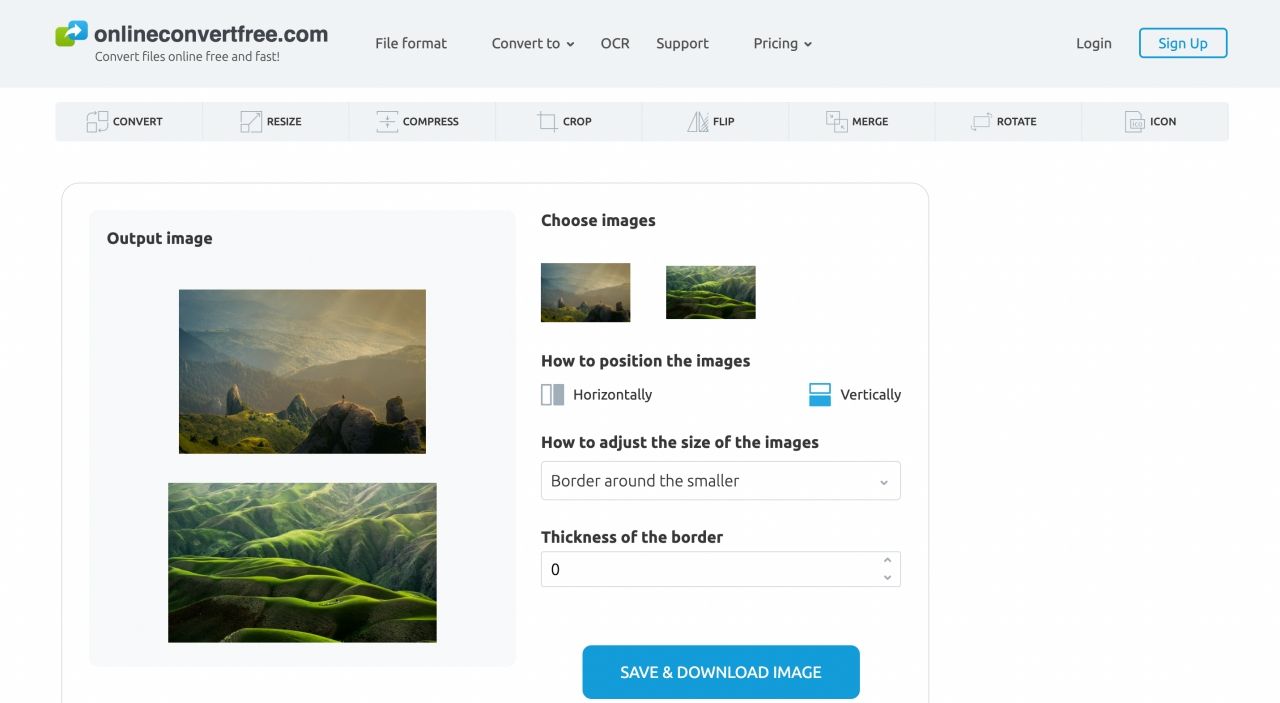A screenshot of the website "onlineconvertfree.com" is displayed, showcasing its main interface for converting files online quickly and for free. The webpage is divided into multiple sections and tabs named "File format," "Convert to," "OCR," "Support," and "Pricing." In the top right corner, there are buttons for logging in and signing up, with the "Sign Up" button highlighted in a blue box for emphasis.

Below this, various tools for image manipulation are listed with corresponding icons, including options for converting, resizing, compressing, cropping, flipping, merging, rotating, and creating icons from images. Two sample landscape images are shown prominently on the page, labeled "Output Image" at the top left. Adjacent to this, on the right, there are smaller thumbnail previews under a header that reads "Choose Images." 

Users can select how the images are positioned - either horizontally or vertically - with the current selection being vertically. Beneath this section, there are settings for adjusting the size of the images via a drop-down menu, which is currently set to "border around the smaller." The border thickness is adjustable, with "0" displayed in the text box. A blue button at the bottom of the section allows users to "Save and Download Image."